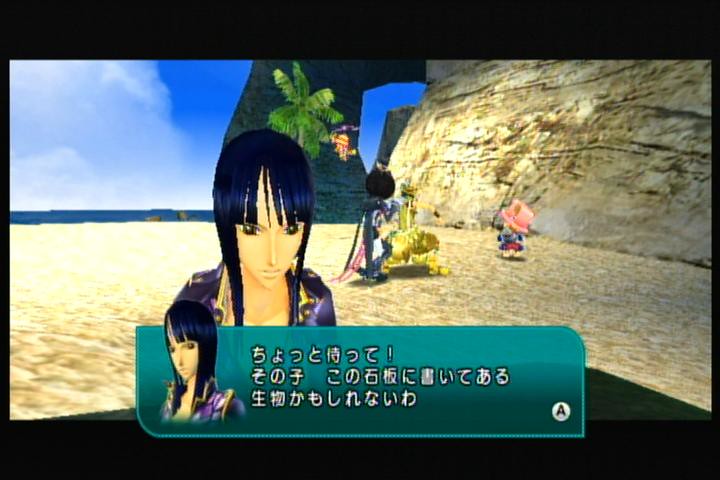This image is a screenshot from a vintage video game, capturing a serene beach scene. The background features a clear blue sky with a few clouds and a distant ocean meeting the horizon in dark blue. A sandy beach with golden sand stretches from the bottom of the frame to the water's edge. To the right, there is a sandy stone structure resembling part of a mountain, with a palm tree standing in front of it. 

In the scene, there are several characters, though most are not clearly visible. One character is tall, and another, shorter one wears a pink hat. A notable character is an anime-style woman positioned directly in the middle, facing the camera. She has sleek, straight blue-black hair with wispy bangs and twin ponytails framing her face, giving her an olive complexion. Her sharp, slanted eyes add to her distinct appearance. This woman is dressed in a purple shirt and is featured in a teal rectangular dialogue box with Japanese text, located at the bottom of the image. Adjacent to this text box, in the right corner, is a letter "A" in black on a white background.

Overall, the screenshot captures a tropical, game-like atmosphere with detailed elements reminiscent of a YouTube video showcasing gameplay.